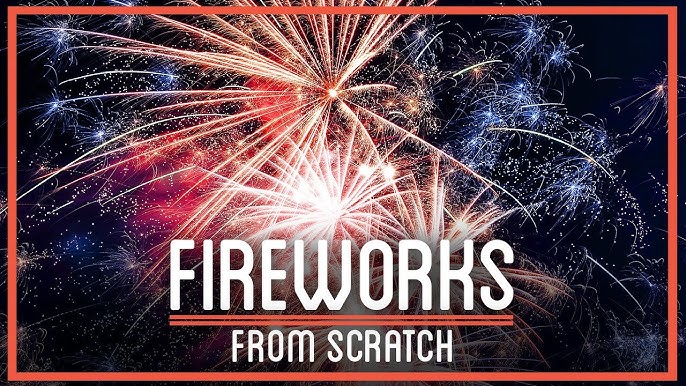This image is a poster featuring a vibrant fireworks display against a dark night sky. The poster is framed by a red border and prominently displays, in bold white letters at the bottom middle, the text "fireworks," underscored by two red lines, followed by the phrase "from scratch." The central part of the image showcases a large, brilliant orange firework explosion that radiates bright lines from a small, intense point. Below this, a more extensive explosion with thicker, white trails dominates the scene. Surrounding these central fireworks are several smaller blue and red explosions, adding depth and variety to the display. The sky behind the fireworks is a deep black or dark blue, enhancing the bright colors. Overall, the fireworks in the middle are predominantly red, orange, and white, with the smaller fireworks around the edges being blue and purple.